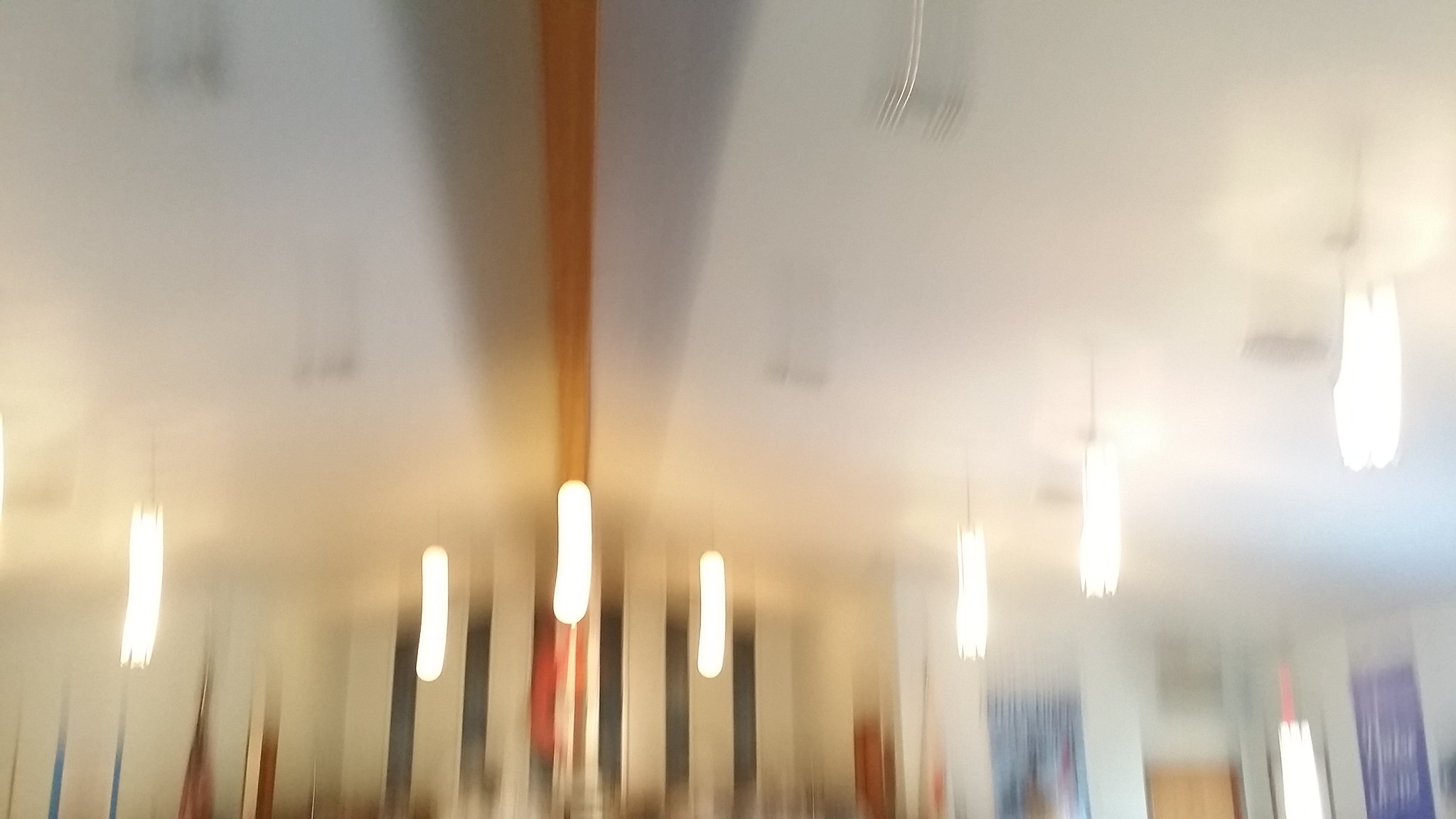The image is an abstract artwork, possibly a painting, characterized by a predominantly gray background with varying shades. At the center-left, there is a prominent brown line, from which a gray, cone-like shape emerges. This shape is wider at the top and narrows towards the bottom. Scattered across the composition are eight distinct, pure white areas that appear to be painted over the original background, creating a striking contrast. The lower part of the image features an assortment of vertical lines in blue and dark blue hues, some faint and others more pronounced, adding a sense of texture and depth. On the right side, the lines transition into rectangular shapes reminiscent of curtains or drapes over windows, primarily in blue, enhancing the abstract and layered nature of the artwork.